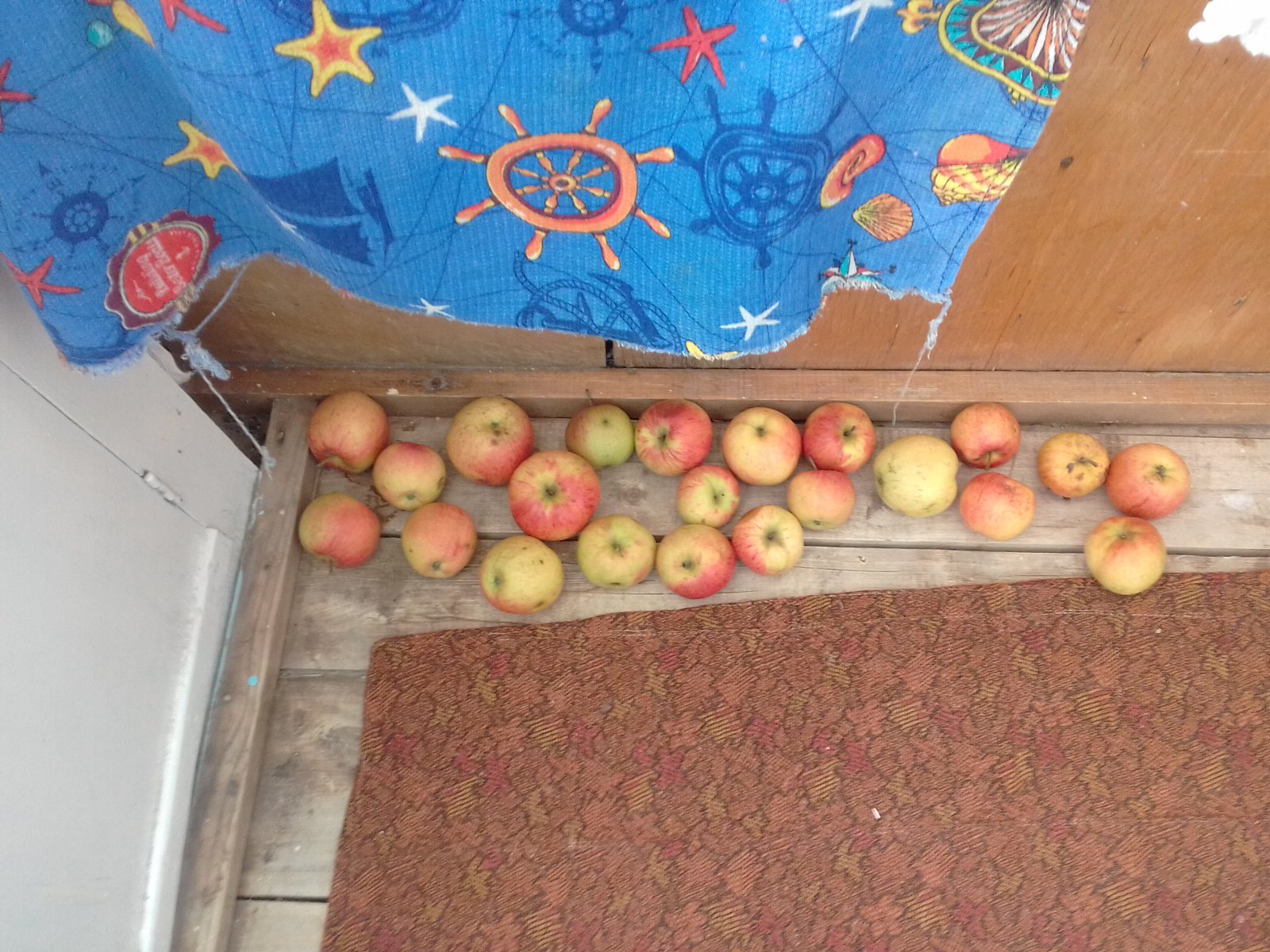In this detailed overhead image, a collection of apples, predominantly red with hints of yellow and green, are scattered on a wooden plank floor. The apples span from the left side to nearly the right side of the image and are surrounded by a reddish-brown carpet, which is slightly angled. To the left, there is a darker and shinier wooden wall or possibly a wardrobe, next to a section of a white wall that includes a door frame with visible hinges. Hanging from the brown wooden surface, there's a large blue cloth decorated with nautical-themed patterns including a ship's wheel, a compass, stars, a rudder, starfish, snails, and sailboats. The scene is brightly lit, and the quality of the photo is very clear, capturing intricate details of the setting.